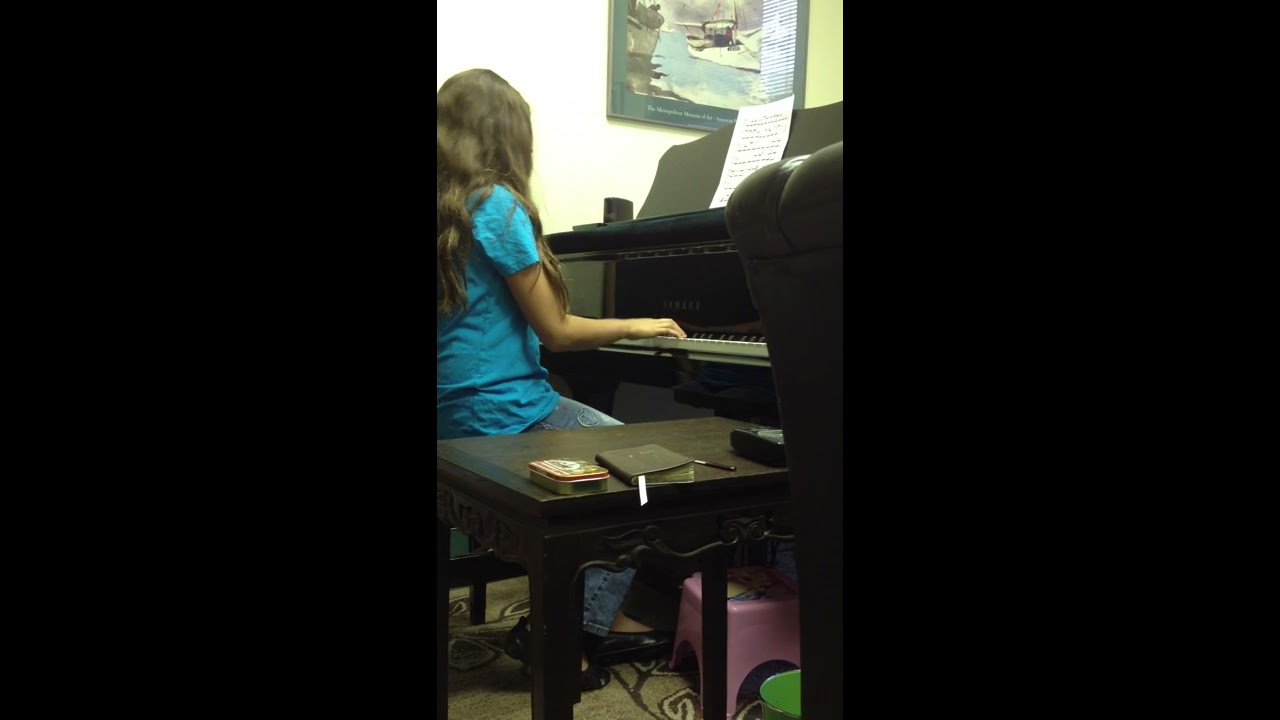The image is divided into three panels, with vertical black bars on the left and right. The center panel features a detailed scene of a person seated at a piano, captured from behind. This individual, likely a woman due to her long, dark brown or brunette hair, is wearing a blue, wrinkled t-shirt and blue jeans. She has on black shoes, visible just slightly. The piano itself is classic and black, with a sheet of music placed on the piano shelf. A wooden table appears in the foreground, holding several items, including a book with a marker, a pen, and possibly a tin. On the right side of the image, a chair obstructs part of the piano. The room's white wall at the back showcases a framed picture, possibly featuring water and white elements, bordered in green. Beneath the piano, a small, pink-colored foot stand or stool with blue, pale yellow, and green protrusions is visible. Additionally, a gold, black, and white rug adorns the floor. There may also be a reflection of Venetian blinds on the left side, suggesting another light source in the room.